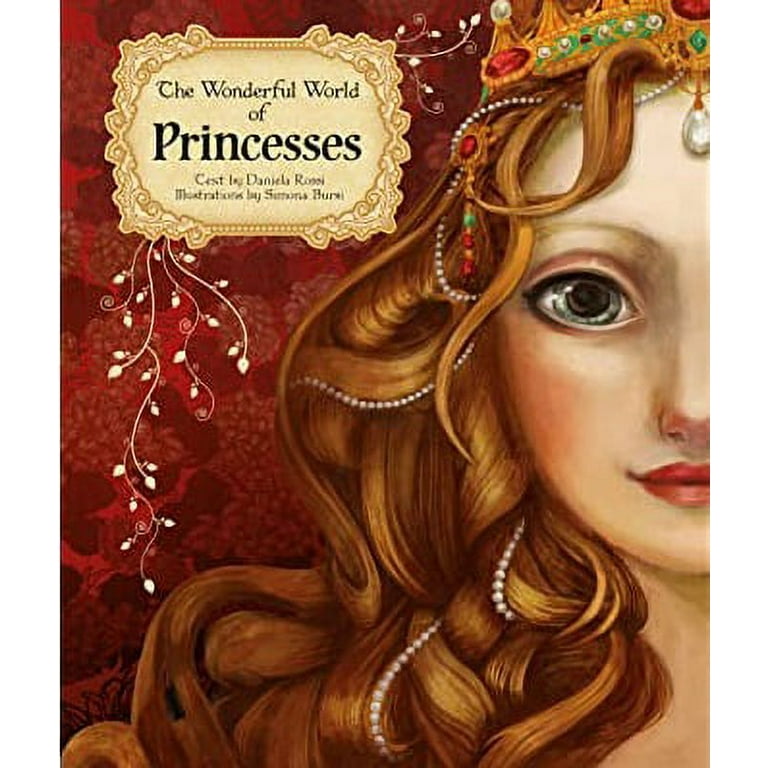The image is an illustration, likely the cover of a book titled "The Wonderful World of Princesses." The title is displayed in an ornate, goldish-yellow box adorned with intricate patterns and white vine-like designs. The cover features a predominantly red background with floral motifs, most visible on the left and middle sections. On the right side, there is a detailed illustration of a princess, showcasing only the left half of her face. 

The princess has long, flowing auburn hair intertwined with white pearls and a slight golden element extending from her crown. Her crown is orange, encrusted with red jewels, white pearls, and some green gems. Her visible features include a large, expressive grey eye, red lipstick, and a serene expression as she gazes forward. The overall composition and details, though slightly blurred, suggest an elegant and dreamy portrayal fitting the book's title.